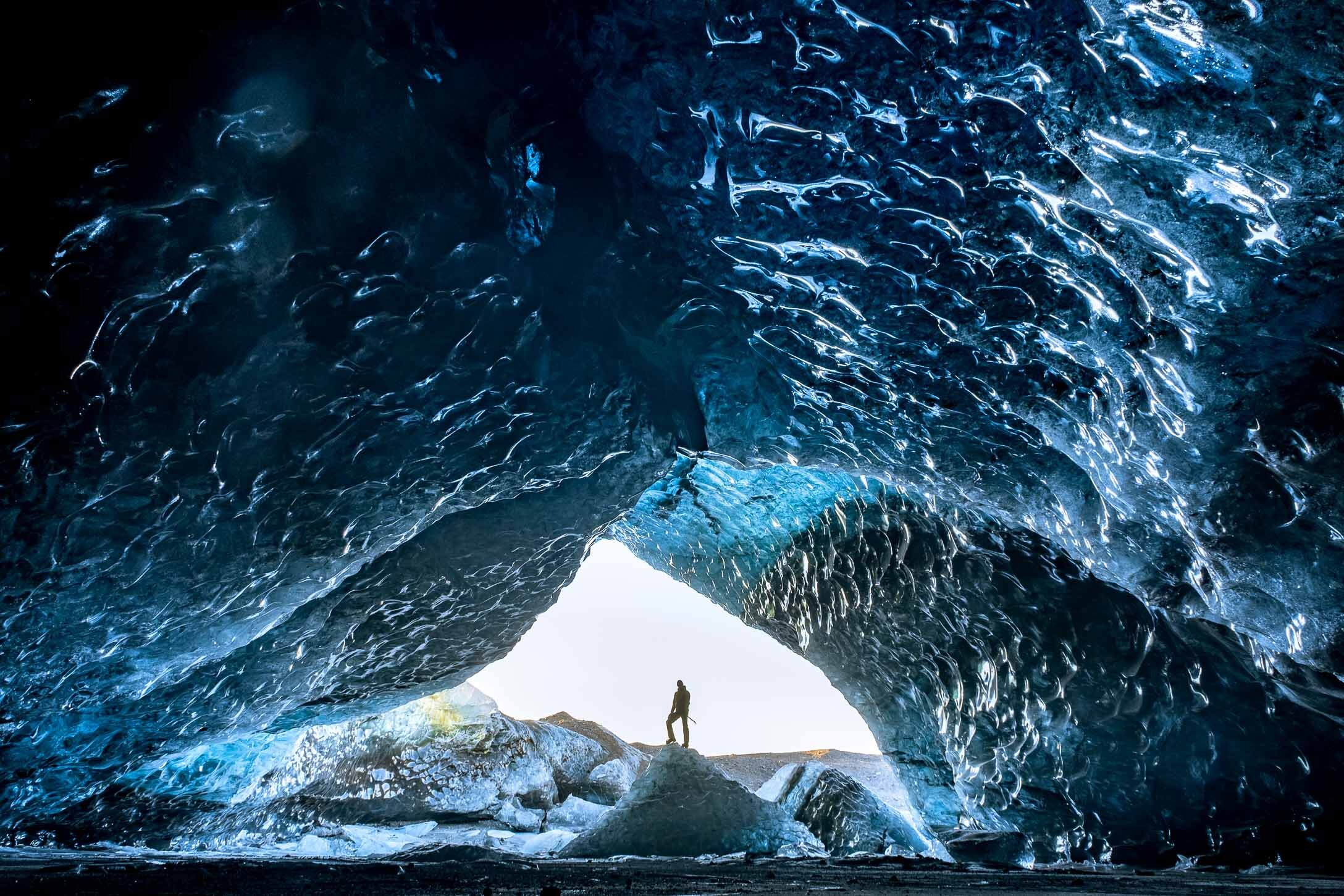The image depicts a striking ice cave interior with rough, porous walls exhibiting an array of dark navy, black, and various shimmering blue tones. The cave forms an impressive, upside-down V shape towards the horizon, where a triangular opening reveals a bright, white sky. Below this scene, dark, almost black waters create a stark contrast. The icy surfaces of the cave are textured with reflections that give off varying degrees of blues and blacks. Amidst this dramatic environment, a silhouette of a man stands on rugged rocks at the cave's edge, poised with one knee up on an iceberg, gazing outward toward the vast expanse. The scene outside the cave appears bright, suggesting daytime, and adds to the overall sense of isolation and grandeur within the icy cavern.